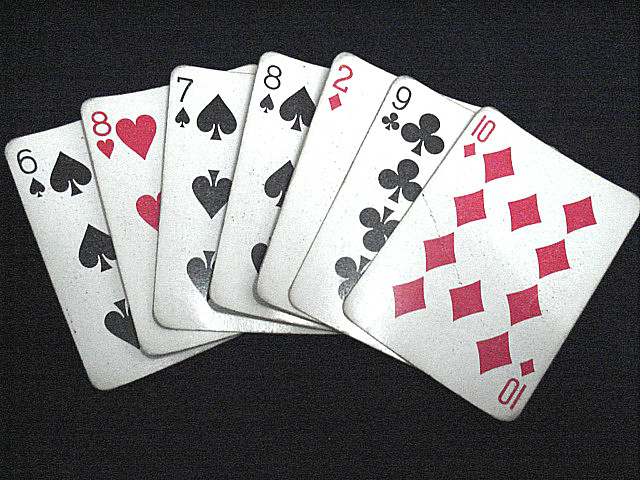This image features a close-up of seven used playing cards from a deck, arrayed in a slightly fanned and arched arrangement against a textured blackish-gray background. From the bottom up, the cards are layered to reveal just a sliver of each, in the following order: the six of spades (black), the eight of hearts (red), the seven of spades (black), the eight of spades (black), the two of diamonds (red), the nine of clubs (black), and the ten of diamonds (red) at the top. The background has shades of gray interwoven, providing a sense of depth and texture. The photograph has a grainy, gritty appearance, with reflections of light visible particularly on the seven of spades and the ten of diamonds, hinting at the worn condition of the cards which bear small black dots and signs of use.